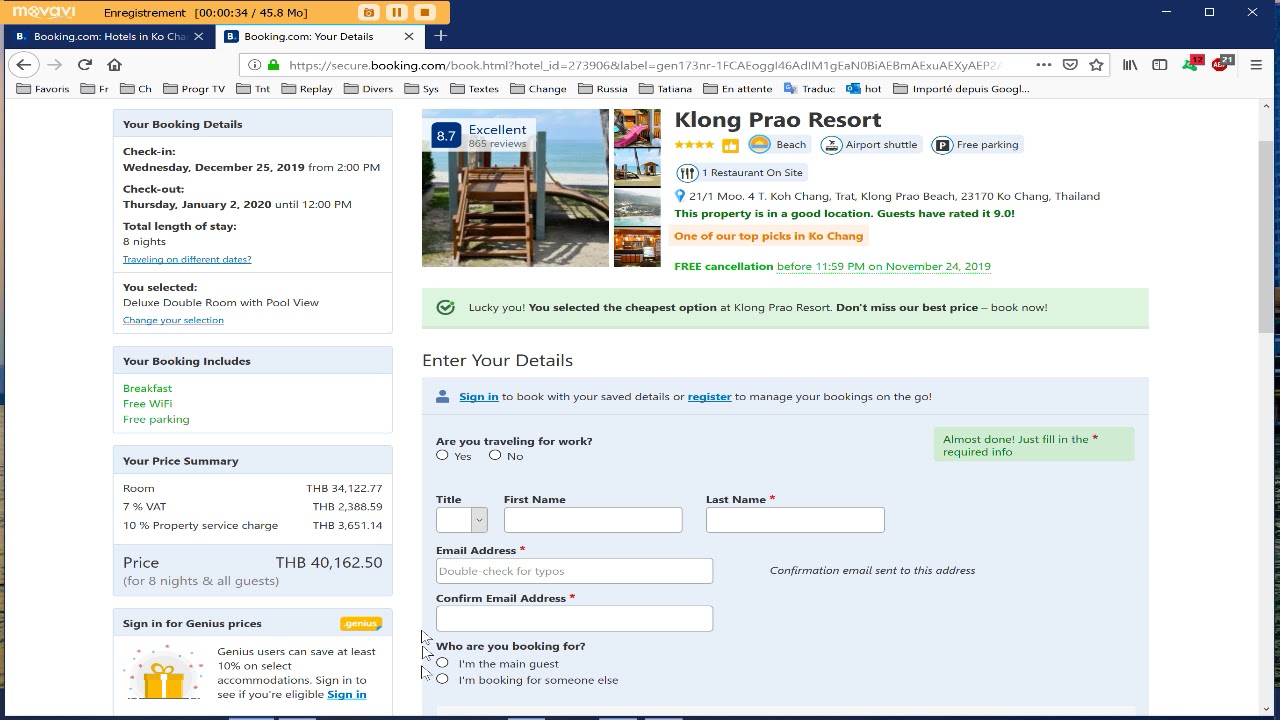Here's a refined and detailed caption for the image:

"A screenshot from a web browser displaying a booking confirmation page on Booking.com. The page is for a stay at Klang Prao Resort in Koh Chang, Thailand. The reservation details show a check-in date of Wednesday, December 25, 2019, and a check-out date of Thursday, January 2, 2020, indicating an eight-night stay. The total cost of the stay is 40,162.5 THB, which includes room value plus 7% VAT and a 10% property service charge. The booking features amenities such as breakfast, free Wi-Fi, and free parking. The resort is described as one of the top picks for Koh Chang, boasting an excellent rating of 8.7. The screenshot includes a photo of a slide with a ladder leading into the ocean, encapsulating the scenic beauty of the resort. The page further includes sections for personal details like title, first name, last name, email, and travel purpose, along with a summary of the booking details and options to confirm the booking."